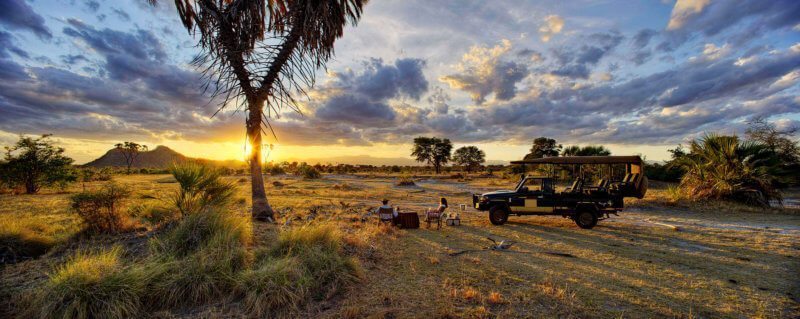In this expansive, panoramic image set at either sunrise or sunset, the bright yellow sun dominates the horizon, its rays reflecting off the clouds ranging in hues from yellow to purple and blue. The sky transitions from these vibrant colors into a pale blue. Prominently in the foreground stands a majestic palm tree with a V-shaped split in its trunk, its leaves framing the glowing sun. The landscape appears to be an African savanna, with sporadically placed trees, a grassy field, and distant mountains receding into the background.

In the mid-ground, a couple sits comfortably on chairs, with a black table between them. Behind the woman, there is a modified truck, possibly used for safari tours, indicative of the adventurous setting. The vehicle appears to blend rugged practicality with passenger comfort, hinting at explorations in remote areas. A bird, possibly a duck, can be seen in the field, adding life to this serene scene.